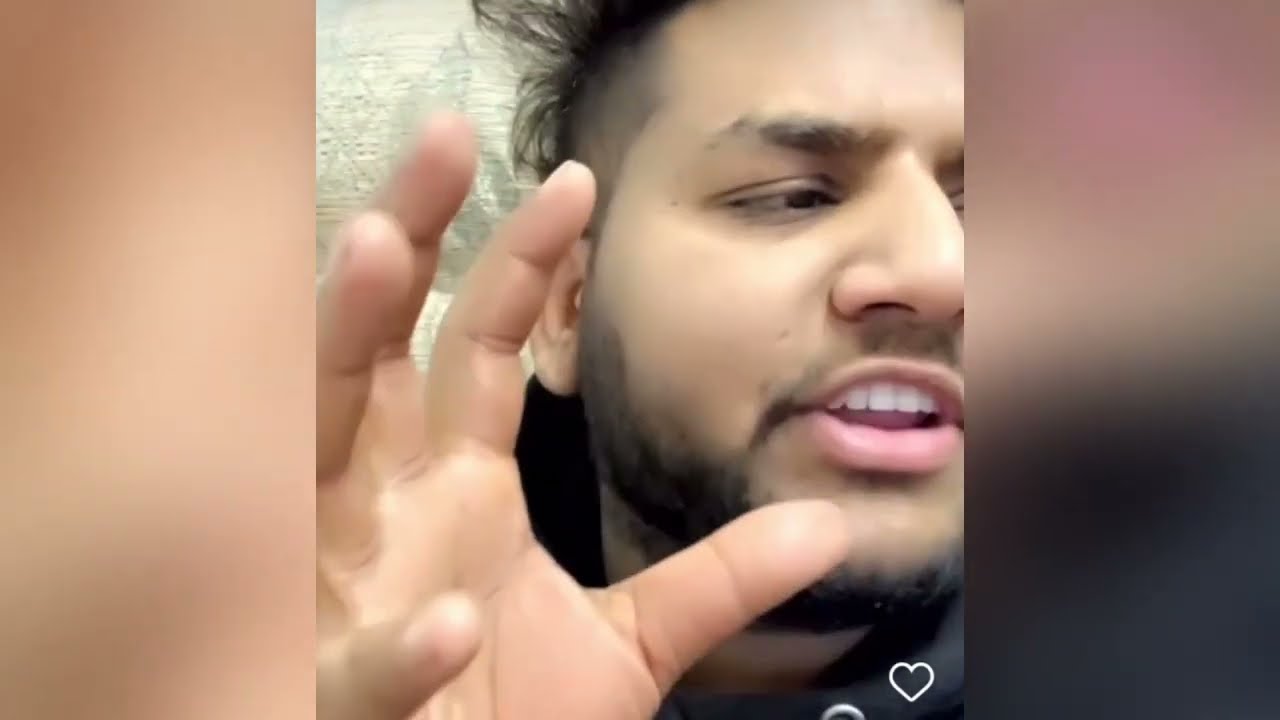In this image, a man with an olive complexion and dark features is prominently centered against a rough, light gray background. His face, which displays dark eyebrows, a light beard, a mustache, and short dark hair, is turned to the right with his mouth slightly open, revealing his teeth and pink bottom lip. His expression suggests he might be talking. He has brown eyes that reflect a thoughtful gaze. His hair, although short and closely cropped on the sides, stands slightly up, casting a shadow on the wall behind him. His left hand is raised beside his face in a claw-like gesture, with closely clipped fingernails and fingers spread apart. Just under his chin, a white heart decal and a small silver circle are visible. Flanking the man, the vertical column on the left is a light peachy blur, while the right column transitions from a rosy hue at the top to black at the bottom, with a peach and beige gradient in between. The man’s attire includes a black shirt that becomes visible partway down his neck.